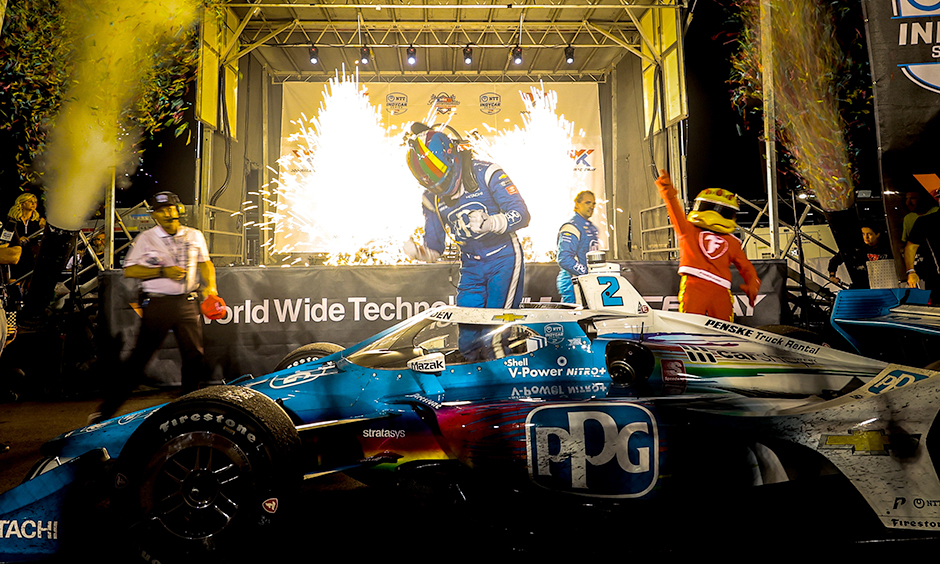The photograph captures a vibrant nighttime scene featuring a celebratory moment in the world of racing. In the foreground, a sleek, low-slung blue race car, emblazoned with the number two and prominent PPG branding, stands distinctive against the dark backdrop. The vehicle's bold design includes other sponsor logos such as Nitrogen Nitro and Shell, and it is adorned with colorful red and yellow stripes along its sides. The racer, clad in a matching blue racing suit with assorted intricate details, wears a multi-colored helmet featuring stripes of yellow, red, green, and purple, obscuring his face as he looks downward, as though preparing for the momentous occasion.

On the right side of the car stands a mascot character, dressed in a striking red outfit with an 'F' on the chest and a bird head boasting sunglasses, likely representing the Firestone brand. Nearby, a team member in a white shirt, black pants, and headset marks the presence of the pit crew, indicating the race's technical and support dimensions.

The backdrop features a grand metal stage adorned with celebratory elements such as confetti cannons and white fireworks erupting into the night sky, signifying a victorious or momentous event. The stage displays a partially obscured banner with the words "worldwide technology," amplifying the global significance of this racing spectacle. Further activity and personnel can be discerned in the background, contributing to the overall lively and jubilant atmosphere of the scene. The image encapsulates the thrill and grandeur of a high-stakes racing celebration.